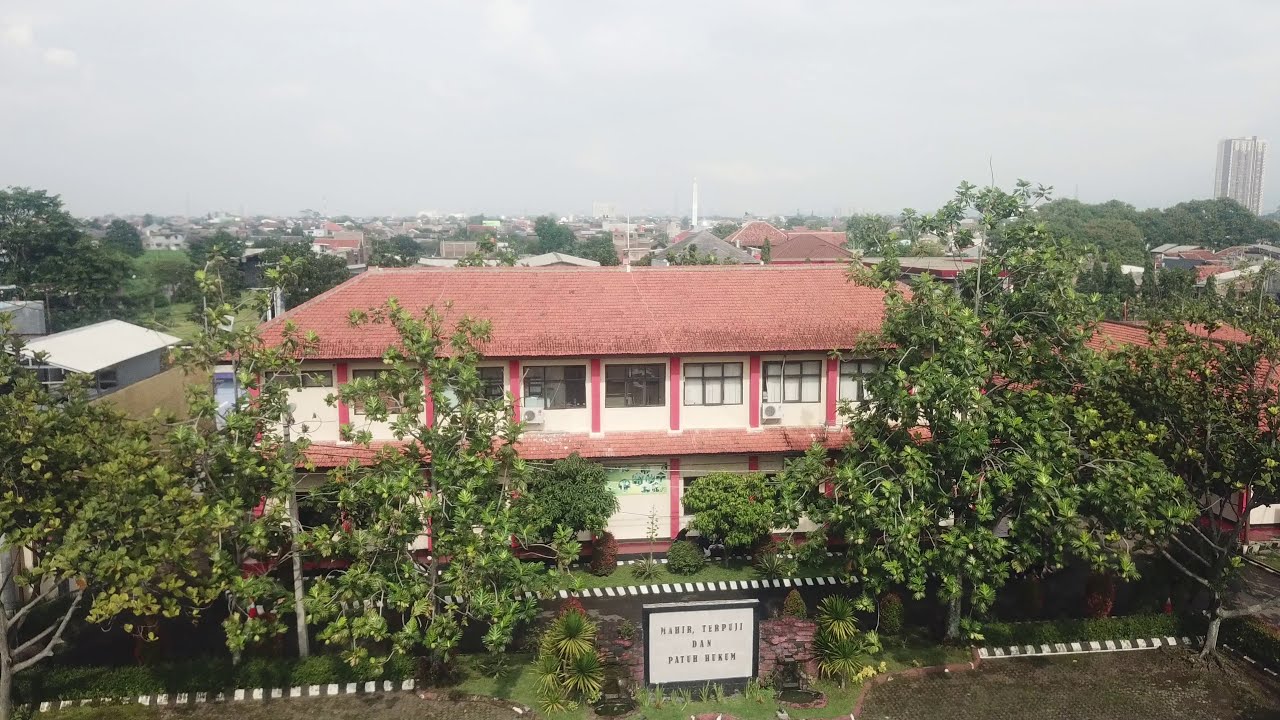A large, two-story building stands prominently in the center of the image, characterized by its bright red roof and accents contrasting with the white walls. Supporting beams, painted a vibrant red, differ slightly in hue from the roof’s brick-red shade. In front of the building are tall, skinny trees adorned with shiny, textured leaves, accompanied by tiny palm trees positioned on either side of a white sign featuring black text that reads “Terpiel Danpadder Decken” or something similar. The background reveals a sprawling cityscape dotted with various buildings and housing, with a notably distant white skyscraper on the top right, standing about 10 miles away. The setting appears to be outdoors during the day, and the surface looks slightly wet, suggesting it might have recently rained. The mix of visible colors includes gray, green, red, orange, black, white, tan, and silver.